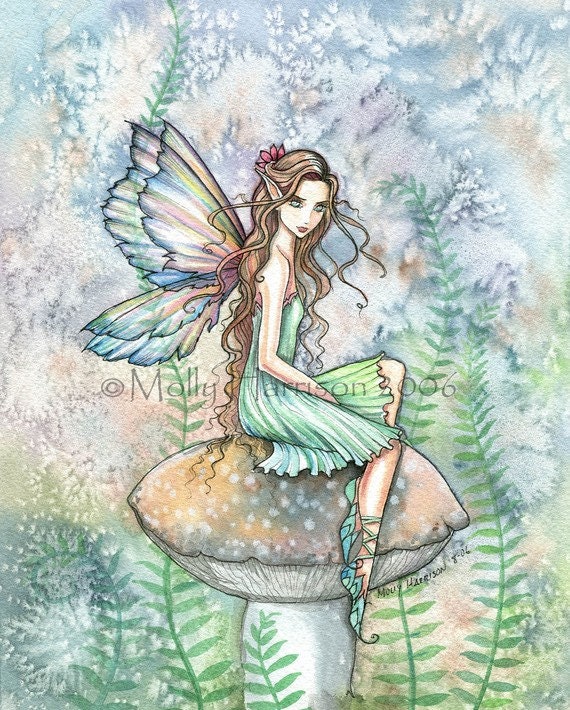This detailed watercolor and ink illustration by Molly Harrison depicts a slender, fairy-like angel with a whimsical, ethereal quality. The fairy, with her distinct pointy elf ears and flowing brunette hair cascading down to her seated position on a large, light brown mushroom with white spots and a white base, exudes an aura of enchantment. She wears a knee-length, pleated turquoise-green dress that leaves her arms and upper chest exposed, paired with matching green or turquoise greenish-blue slippers with delicate straps wrapped around her ankles, almost like high heels. Her translucent, jagged butterfly wings shimmer in soft hues of blue, green, white, yellow, and turquoise, providing a striking contrast against the dreamlike, pale blue and white cloudy background.

The fairy's striking green eyes and slight pink lipstick accentuate her delicate, light complexion. A subtle red ribbon adorns her hair, adding a charming touch to her overall appearance. She is surrounded by vibrant green plants and fern branches that sprout from the base, adding to the predominantly green theme that gives the image an Irish or woodland elf motif.

The artwork is exquisitely detailed, and two signatures, "Molly Harrison" and "Moe Harrison 806," can be seen, identifying the talented artist behind this enchanting scene.